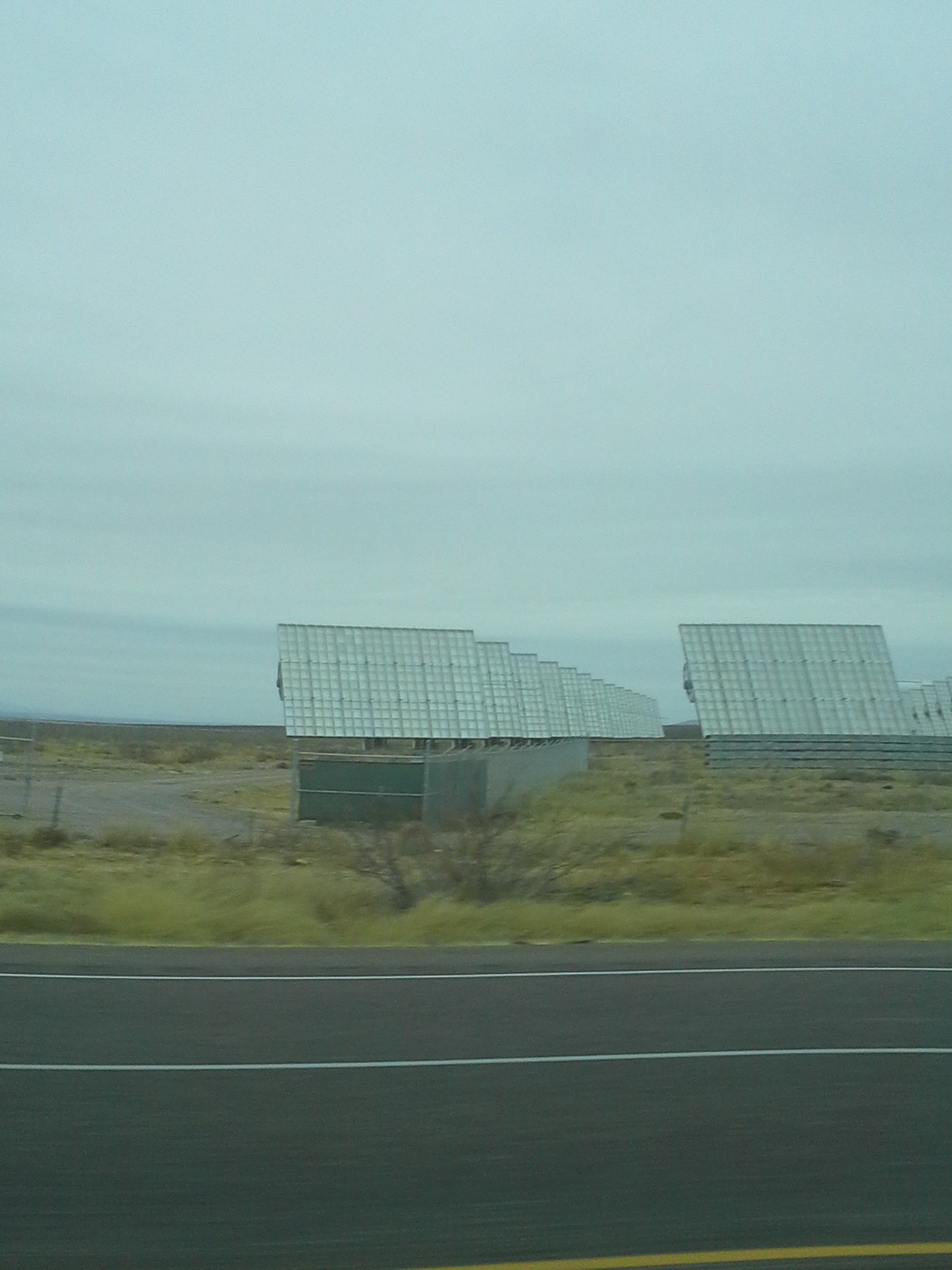In this outdoor photograph taken in broad daylight under an overcast sky, we observe a muted blue-gray expanse overhead with pale, wispy clouds near the horizon. The lower third of the image features a clean, well-maintained highway marked with a central white line and a partial yellow line along the bottom right corner. Across the road, roughly a third of the way up, a patch of low grass and sparse weeds extends towards a fenced-off area.

Beyond the fence, several buildings with slanted, pale blue roofs are visible, their checkerboard-like sections suggestive yet not conclusively identifying them as solar panels. These structures are aligned in rows, angled facing the right of the image, and appear aged or potentially out of use. To the left of these buildings is a smaller, paved or gravel road leading away from the main highway. In the background, the terrain transitions into more brush and grass, devoid of trees or significant vegetation. Overall, the scene depicts a secluded, possibly industrial or abandoned area under a hazy, subdued daylight.